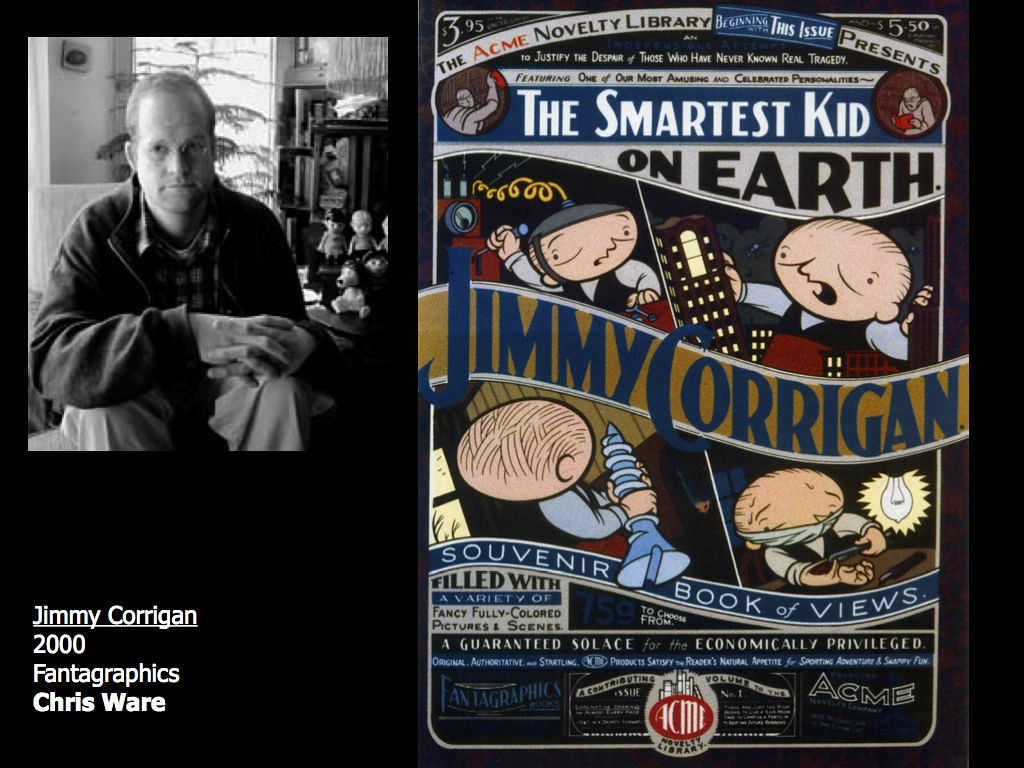This image is a detailed poster for "The Acme Novelty Library," presenting "The Smartest Kid on Earth," Jimmy Corrigan, created by Chris Ware and published by Fantagraphics in 2000. The central part of the poster features a photograph of a man, possibly Jimmy Corrigan or Chris Ware, sitting in a chair inside a house. He is dressed in a jacket with a checkered shirt, glasses, and has his hands clasped together. In the lower left-hand corner, it reads "Jimmy Corrigan, 2000, Fantagraphics, Chris Ware."

The poster describes it as a "Souvenir Book of Views," which is filled with a variety of fully colored picture scenes providing guaranteed solace for the economically privileged. The narrative hints at Jimmy Corrigan, who is portrayed as a cartoon character engaged in MacGyver-like activities, inventing gadgets and coming up with clever ideas. The design in the lower portion features a red background with white lettering that reads "Acme," accompanied by a cartoon drawing of a person holding various items: a bomb, a building, a screw, and handcuffs being removed. This visually represents the ingenuity and imaginative world of Jimmy Corrigan as crafted by Chris Ware.